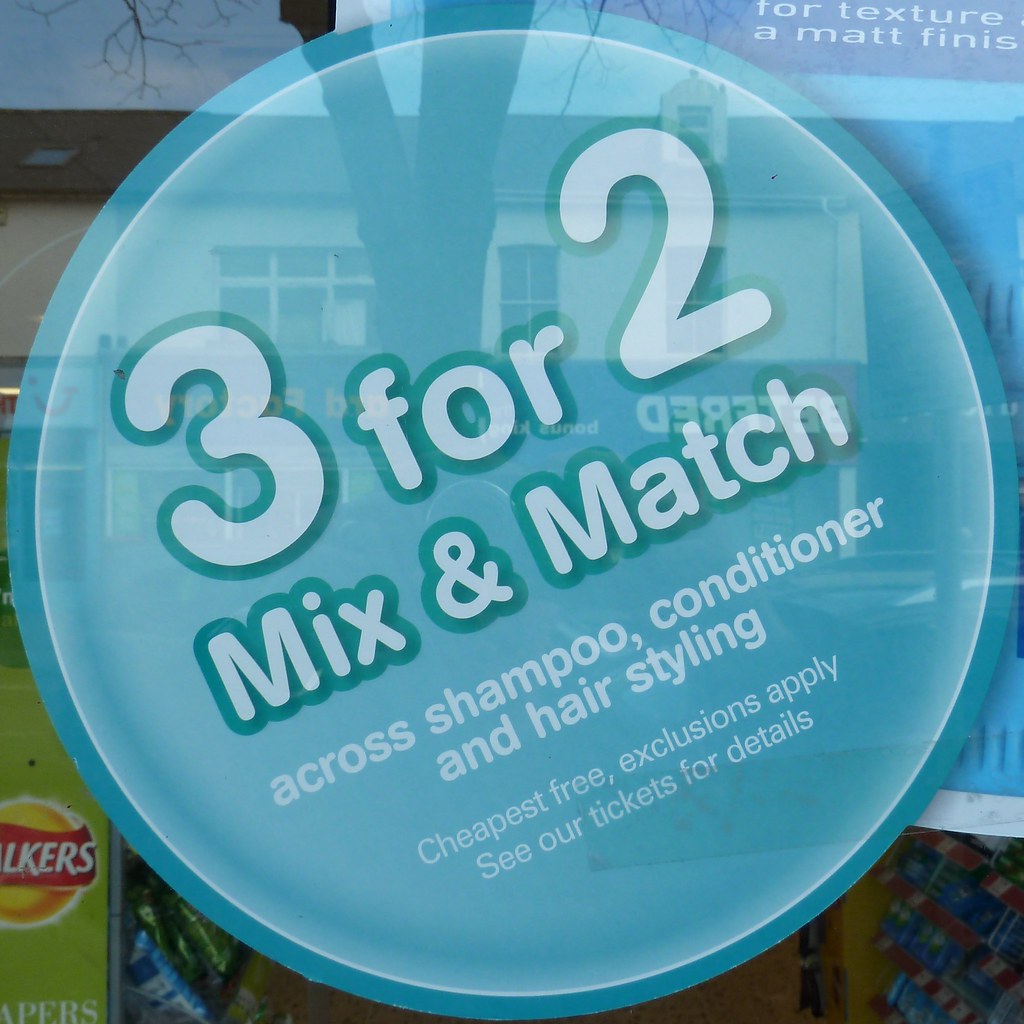The vibrant daytime image appears to be an advertisement prominently displayed in a store window, with a clear reflection of a two-story building and possibly the photographer themselves. The main feature is a light blue circular sign, slightly tilted 45 degrees, centrally positioned with an enticing promotion in bold white lettering that reads, "Three for Two, Mix and Match." Below, smaller white text elaborates, "Across shampoo, conditioner, and hairstyling. Cheapest free, exclusions apply, see our tickets for details." Accentuating the sign, some letters and numbers are outlined in green. Additionally, in the upper right corner, partially obscured, the text promises "For texture and a matte finish," although the word "finish" is cut off. In the image's bottom left corner, there is a sandwich board highlighting the UK chip brand "Walkers." The setting captures the natural brightness of the day, providing a well-lit, clear view of the advertisement.